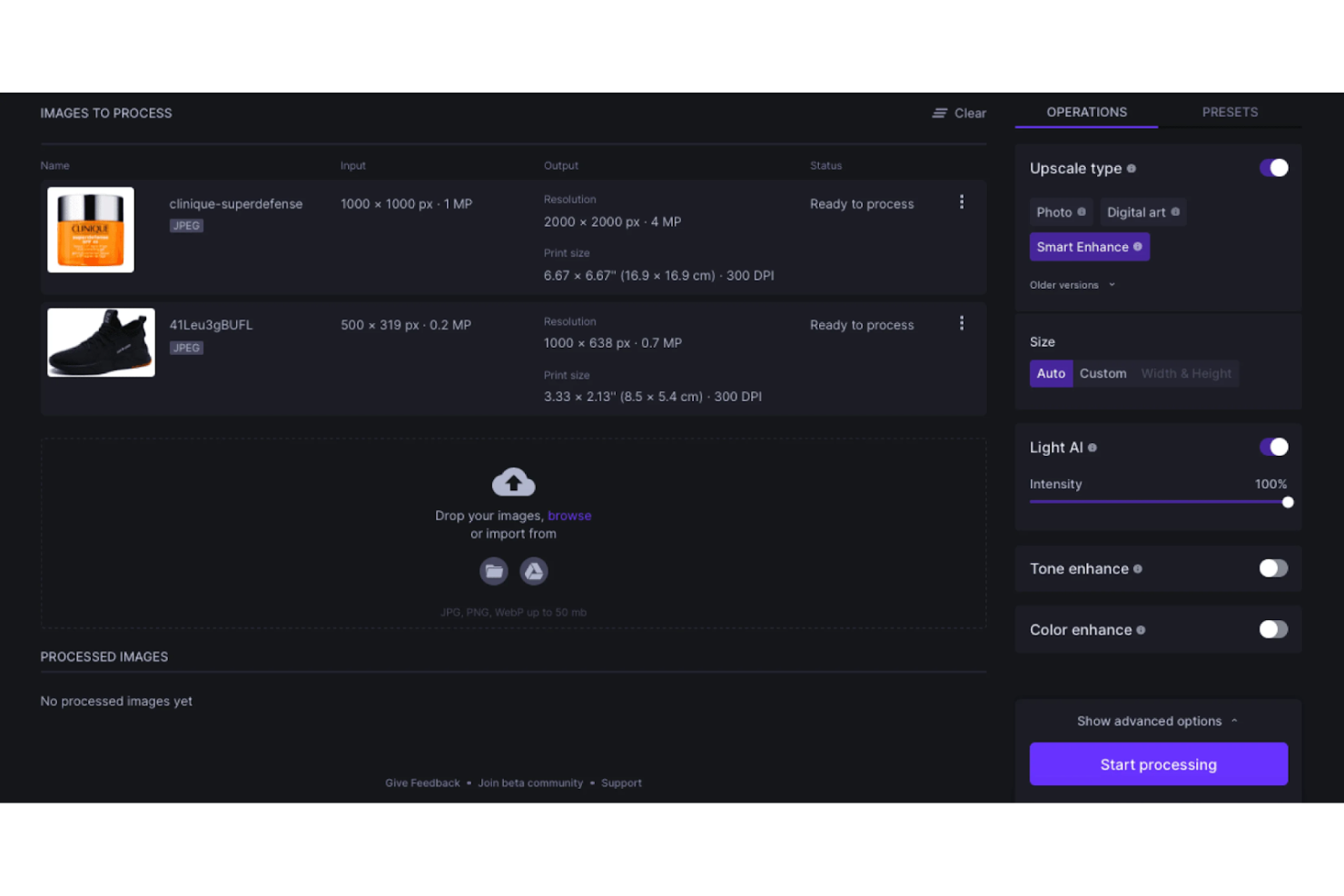Here is a detailed and cleaned-up descriptive caption for the image:

---

The screenshot displays an image processing software interface. The main section features a table with columns labeled "Name," "Input," "Output," and "Status." The first entry in the table is for an image named "Clinique Super Defense.JPG" with an input resolution of 1000 x 1000 pixels (1 megapixel). For the output, the resolution is set to be 2000 x 2000 pixels (4 megapixels), and the status is marked "Ready to Process." Adjacent to this status, there are three ellipsis marks indicating additional menu options.

The second entry is an image of a sneaker labeled "41_LEU_3G_BU_FL.JPG" with an input resolution of 500 x 319 pixels (0.2 megapixels). The output resolution is specified to be 1000 x 638 pixels (0.7 megapixels), with the status also marked "Ready to Process." The printed size for this image is noted as 3.33 x 2.13 inches (8.85 x 5.41 cm) at 300 DPI, while the Clinique image above is sized at 6.67 x 6.67 inches (16.92 x 16.92 cm) at 300 DPI.

Below the table, there is a prompt to "Drop your images, browse, or import from," along with icons for JPEG, PNG, among others. A nearby folder and recycle bin icon are labeled "Processed Images," but currently, it states "No Processed Images Yet."

On the right side of the interface, the "Operations" tab is highlighted, next to another tab for "Presets." Within the operations section, there are options for "Upscale Type" (with "Photo" and "Digital Art" sub-options) and "Smart Enhance." Other settings include "Older Versions" with a dropdown menu, "Size" with "Auto" selected, and options for custom width and height. The "AI Intensity" is set to 100% and turned on, while "Tone Enhance" and "Color Enhance" are turned off. There is also a collapsed section for "Show Advanced Options."

At the bottom-right, a prominent purplish-blue button labeled "Start Processing" in white text awaits the user’s action.

---

This caption provides a comprehensive and organized description of the image and its elements, allowing readers to understand the interface without visual cues.